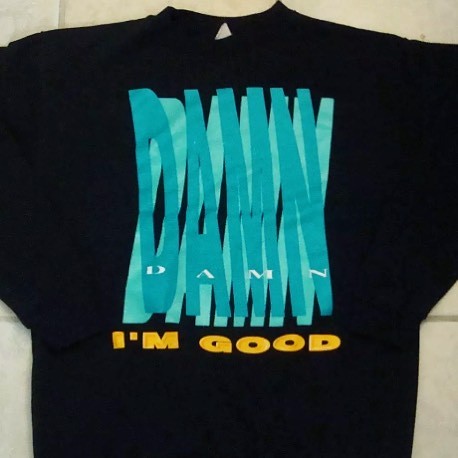A black t-shirt is meticulously laid out on a surface adorned with white tiles. The shirt features a captivating graphic design. The word "Damn" is prominently displayed in large, elongated blue letters that tilt from left to right. Each letter casts a lighter blue shadow that tilts in the opposite direction, creating a dynamic visual effect. Directly beneath each of these larger letters, "D-A-M-N" is replicated in smaller white text. Below this striking arrangement, the phrase "I'm good" appears in bold yellow letters, perfectly centered on the shirt. The t-shirt has a rounded collar with a small portion of the white clothing tag visible at the top, adding a subtle touch of detail to the garment's presentation.